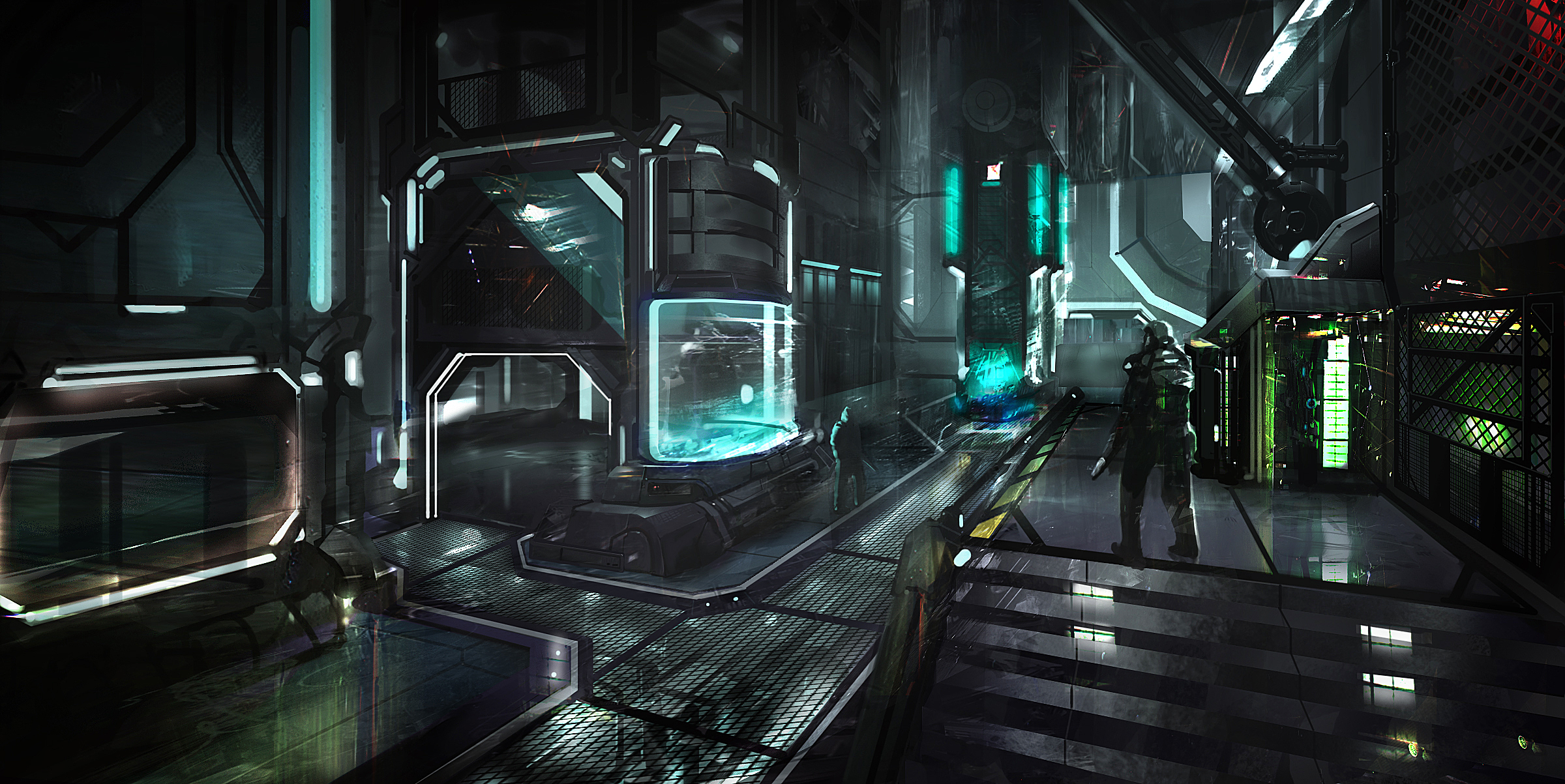The image depicts a dark, futuristic setting that could be from a video game or a detailed artwork, featuring a large, dimly lit room that evokes a factory or spaceship environment. The floor is composed of metal grates with light filtering through from below, enhancing the atmospheric effect. The wide steps leading upwards appear to be made of translucent material, possibly glass, with neon lighting integrated into the walls, casting shades of blue and green.

At the top of the stairs stands a character dressed in a dark suit, potentially with a helmet, holding an indistinguishable object, which might be a weapon. The central focus of the scene is occupied by a large, glowing glass area on the left, which reflects the ambient lights and has a blue-green tinge. The background reveals a larger room illuminated by neon lights, providing depth to the setting. The entirety of the space is predominantly grey with accents of blue and green neon, emphasizing the industrial, high-tech atmosphere.